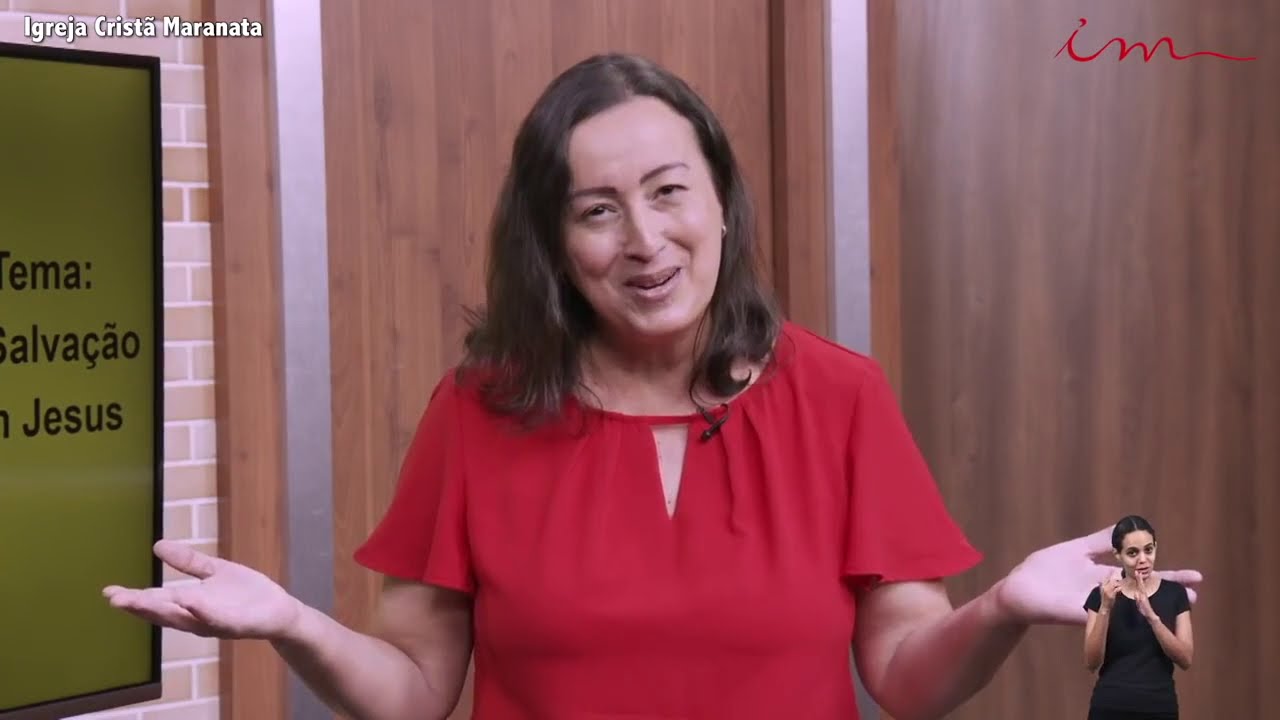The image appears to be a scene from a TV show or a presentation, featuring a woman centrally located and prominently positioned in a wide rectangular frame. She has white skin and short brown hair, wearing a flowy red dress shirt and smiling, with both hands out and palms facing up, suggesting she is speaking or presenting. In the background, there is a smooth wooden wall that transitions from light brown to gray with silver vertical rectangles at the corners, adding a touch of modernity to the setting. On the left side, a lighter brown brick wall features a green poster with a black frame, displaying the words "Tema Salvação Jesus." In the bottom right-hand corner of the image, there is a smaller insert of another woman with light brown skin and a black shirt, possibly interpreting the presentation into sign language. Both the central figure and the smaller figure contribute to a sense of engagement and inclusivity in the presentation.